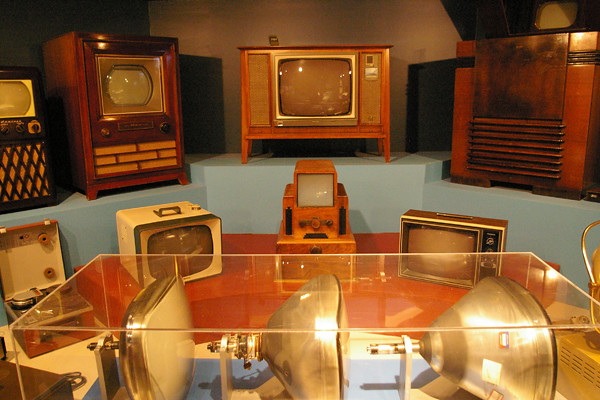The photograph depicts a meticulously arranged museum exhibit showcasing a range of retro television sets, likely from the 1940s, 1950s, and possibly some from the 1970s. The exhibit features an array of console TVs, primarily housed in medium to dark brown wood frames, such as walnut and mahogany, alongside some units in white plastic casings. The television models vary in size, with screen dimensions as small as 14 inches, and some up to 24 or 26 inches. These sets are displayed on built-in countertops and specially designed display shelves, organized at different elevations along the wall. Prominently in the center, there is a large glass case enclosing three substantial bulbs facing to the right, suggestive of an important and delicate piece of television technology from the era. This exhibit not only highlights the evolution of television design but also emphasizes the Americana style prevalent during these decades.